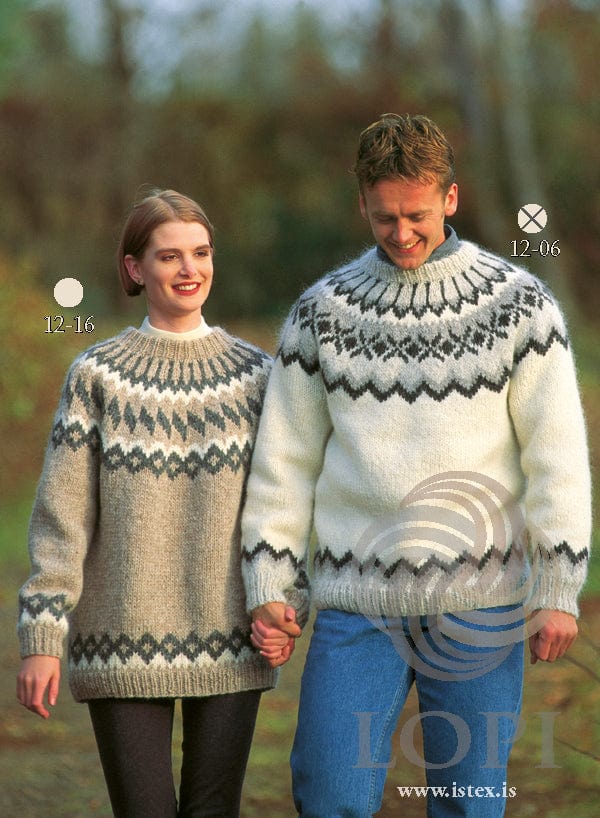This is a photograph of a couple, seemingly in an advertisement for sweaters, walking hand in hand on a trail in a wooded area during early fall. The woman on the left, with brown hair and a smile on her face, is wearing a bulky, oversized wool sweater in shades of tan, dark green, and light tan, featuring intricate designs of feathers, zigzags, and diamonds. She also wears black dungarees. Beside her is a white dot with the numerals "12-16." The man on the right, looking down with a smile, has blondish-brown hair and is dressed in a similarly bulky white, black, and gray sweater displaying patterns of feathers, X's, diamonds, and zigzags. He pairs it with a cream-colored mock turtleneck and blue jeans. Next to him is a white dot with the numerals "12-06." Both sweaters appear to be from the brand "LOPI," with their website www.istex.is faintly visible at the bottom. The couple is set against a blurred backdrop of trees and shrubs, enhancing the cozy and serene autumn atmosphere.